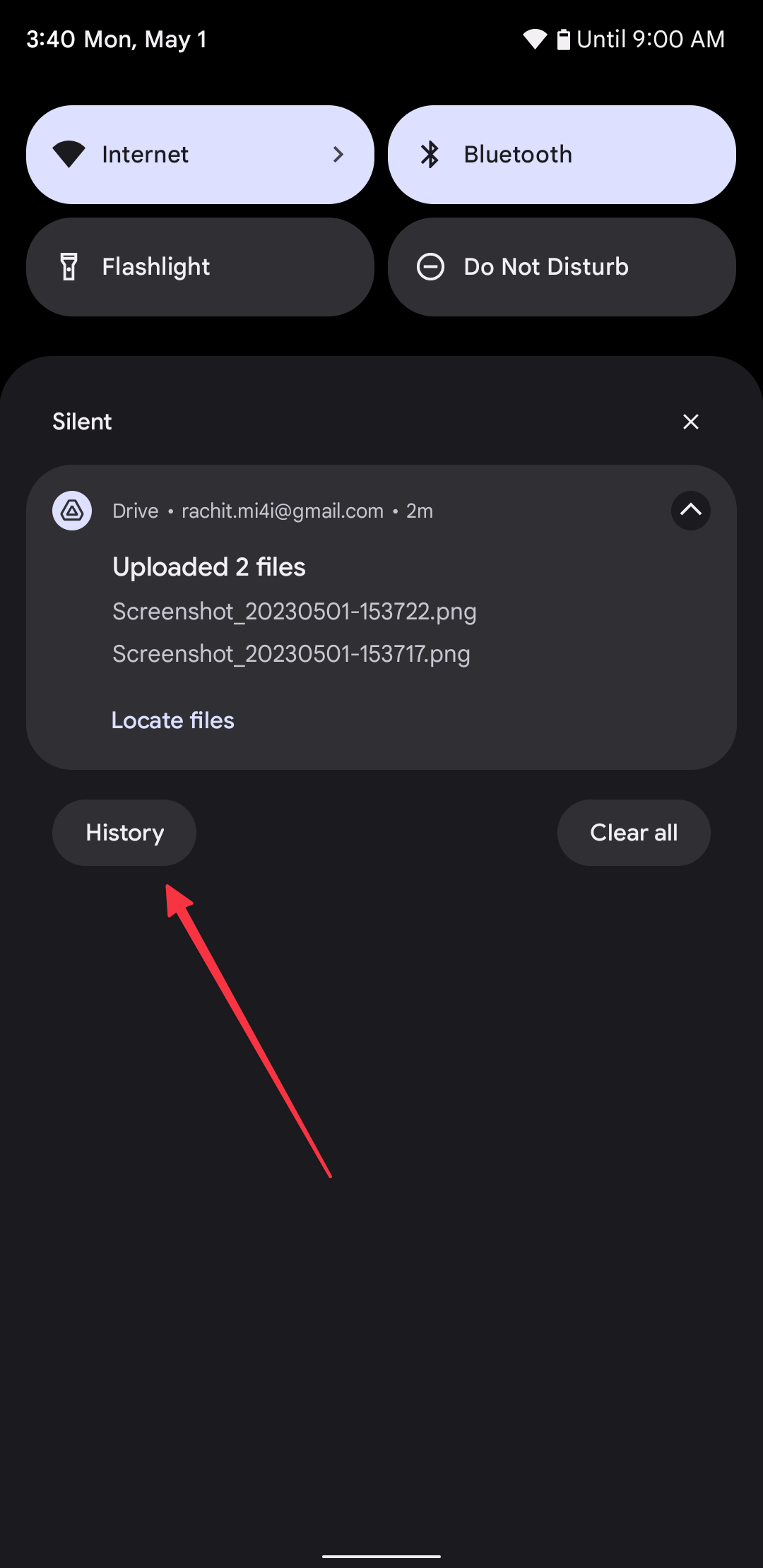This is a detailed screenshot of a phone interface with a black background. At the top left corner, the time is displayed as 3:40, alongside the date, Monday, May 1st. To the right, various icons are visible, including Wi-Fi, battery indicator, and a notation indicating "until 9 a.m."

Below these icons, there are four oval-shaped buttons arranged in a horizontal line. The first two buttons are light blue and labeled "Internet" and "Bluetooth," while the next two are dark gray and labeled "Flashlight" and "Do Not Disturb." Each button features corresponding icons next to the text. 

Beneath these buttons, the word "Silent" appears in white text, accompanied by an "X" icon on the right-hand side. Further down, a pop-up notification displays the email address "drive.reachit.mi4e@gmail.com" with a timestamp of two minutes ago. Adjacent to this, there are triangle and circle icons, indicating that two files have been uploaded.

The notification details show the names of the two uploaded screenshots, accompanied by an option labeled "Locate files." Below the pop-up box, there are two buttons: "History" and "Clear All." A prominent long red arrow points upwards towards the "History" button from the bottom of the screen.